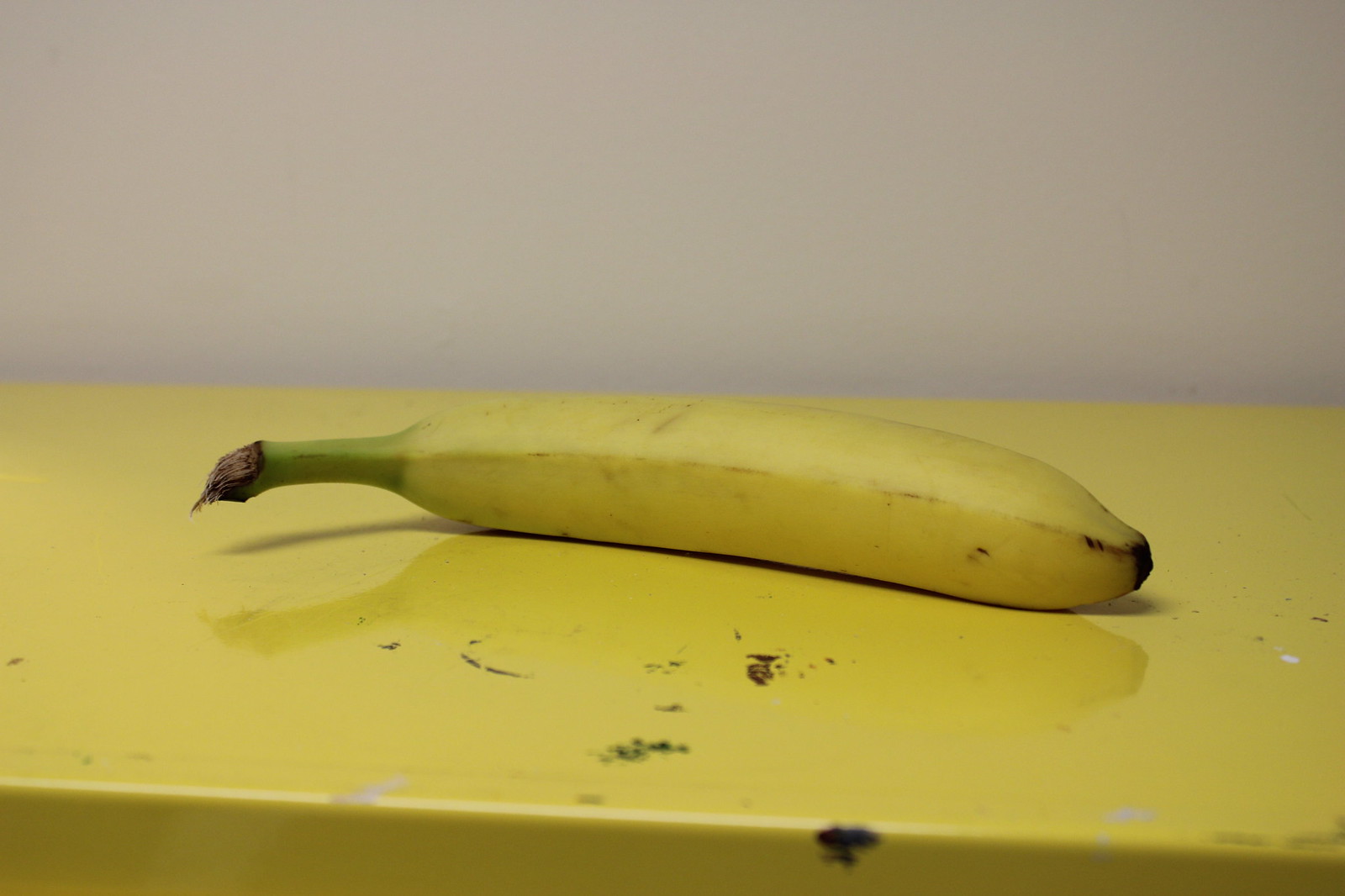A vibrant color photograph captures a single ripe banana resting on a yellow enamel-painted metal surface. The banana, predominantly yellow, shows signs of ripeness with small brown spots and slightly browning edges. Its stem remains distinctly green, indicating its freshness. The surface beneath the banana mirrors its color almost perfectly, albeit with visible wear and tear: brown scratches, scuffs, and areas of rust where the yellow enamel has chipped away. The smooth, glossy finish of the metal creates a faint shadow of the banana, adding depth to the composition. Behind this setup, a plain beige wall serves as a neutral backdrop, highlighting the contrast and similarities between the banana and its resting surface. The banana is positioned side profile, extending horizontally, drawing the viewer's eye along its length and the subtle details of its texture and the aged surface beneath it.